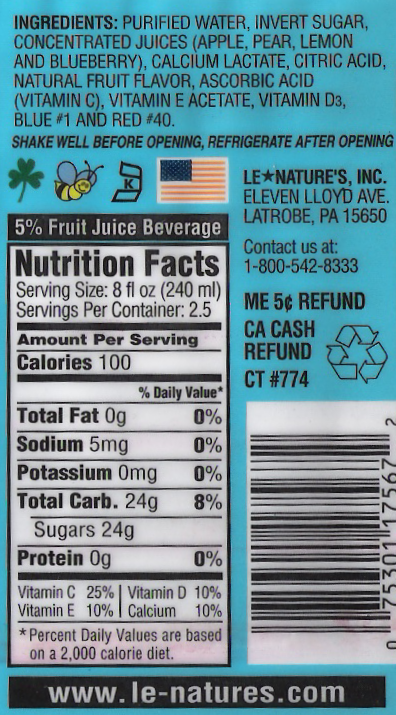Here is a cleaned-up and detailed caption based on the given information:

---

This image showcases the back label of a juice beverage from Lay Natures Inc. The label provides a comprehensive list of ingredients, including purified water, invert sugar, concentrated juices, calcium lactate, citric acid, natural fruit flavor, ascorbic acid (Vitamin C), vitamin E acetate, vitamin D3, Blue No. 1, and Red No. 40. Nutritional information is clearly outlined, ensuring transparency about the beverage's content.

The label includes specific instructions for use: "Shake well before opening." Post-opening, the beverage should be refrigerated to maintain freshness. 

Symbols are prominently displayed, including a clover, a bee, a kosher certification mark, and an American flag, likely indicating the product's manufacturing origin in the USA and possibly its adherence to specific dietary guidelines.

To the right of the label, the company name and contact information are given: Lay Natures Inc., located at 11 Lloyd Avenue, Latrobe, Pennsylvania, 15650. The label also lists a customer service phone number and features a barcode with an associated barcode number.

At the bottom of the label, the company's website is provided, offering consumers an avenue for further information or inquiries about Lay Natures Inc.'s range of products.

---

This detailed caption highlights the various elements present on the juice beverage label, giving a clear and informative overview.